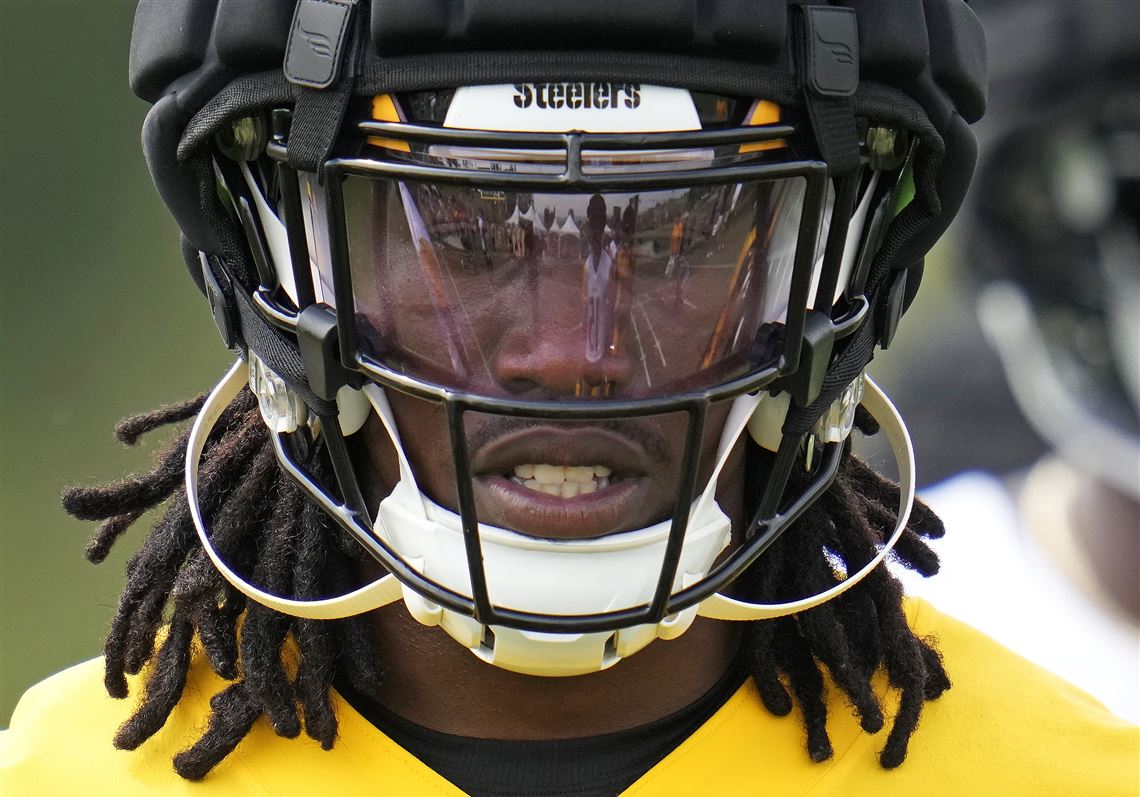This detailed close-up photograph captures a football player from the Pittsburgh Steelers during practice. The player, identified as an African American man with long braided hair and a short mustache, dons a yellow practice jersey over a black shirt. His helmet, featuring a black protective cover, prominently displays the Steelers logo and includes a clear visor that reflects the surrounding players. His mouth is open, revealing his teeth, and he wears a white chin strap that is securely fastened. Above his eyes, the helmet has additional cushioning to mitigate impact. The background, although blurry, shows a player in a white jersey alongside some greenery, indicating an outdoor practice setting. The focused intensity on his face suggests he is mid-action or in a moment of concentration.